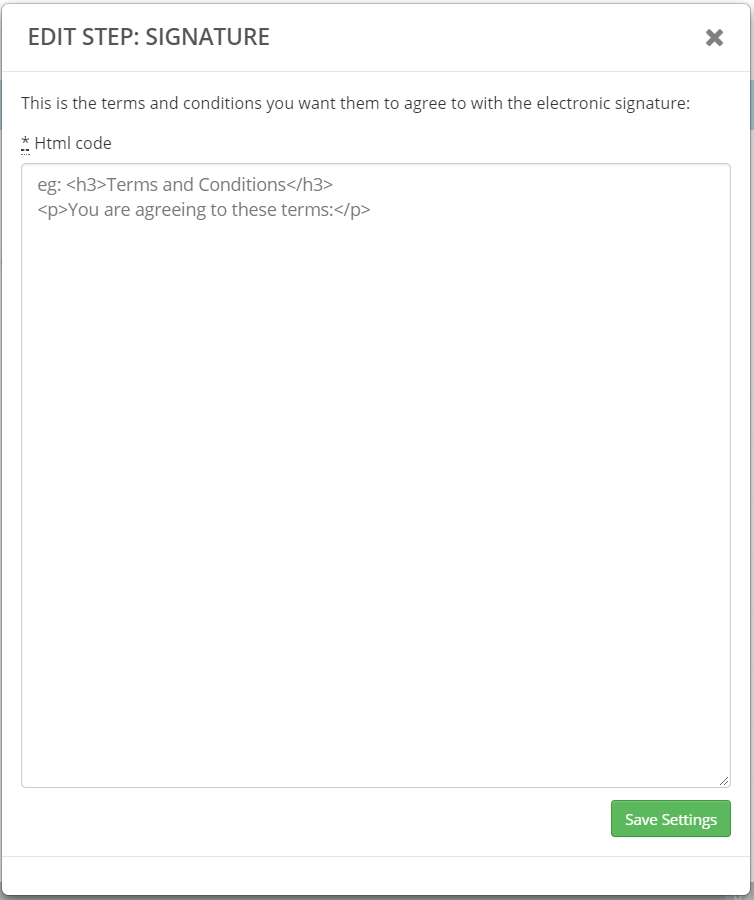This image features a minimalistic webpage that highlights the process of capturing an electronic signature for terms and conditions. The HTML code snippet displayed demonstrates how the page is structured, specifically focusing on the section where users must agree to the terms. The message reads, "You are agreeing to these terms and conditions," with a clear call-to-action button labeled "Save Settings." This represents page 3 of the example walkthrough, detailing the crucial step of securing user consent through a digital signature.